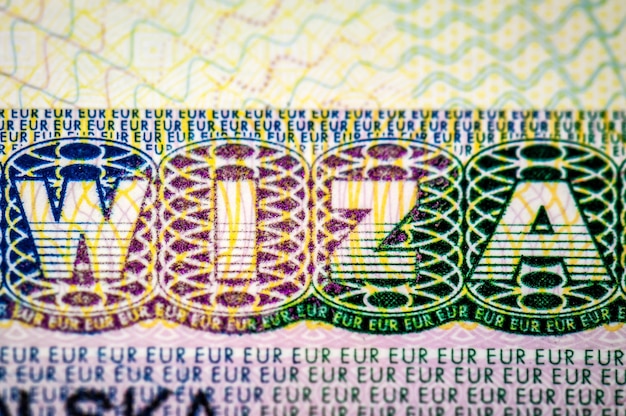This image showcases a vibrant and complex design centered around a logo with the letters "WIZA." The background features a multi-wave pattern with overlapped concentric squiggly lines in shades of yellow, purple, green, and blue, creating a dynamic and colorful telegraph-like appearance. In the upper right corner, a wider blue wave pattern stands out. The borders at the top and bottom of the image consist of four lines each, containing the repeated text "EUR EUR EUR EUR" in various gradients of blue to green. The central focal point of the image is the "WIZA" logo, with each letter enclosed in a cylindrical shape embellished with blue, purple, and green designs. The overall color palette includes dark blue, yellow, cranberry, deep green, and lavender accents, adding to the intricate and layered visual effect.